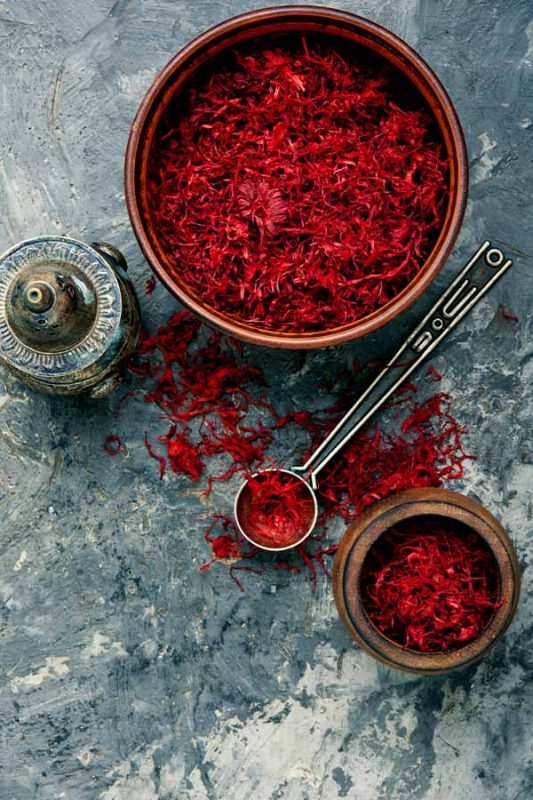The image captures a richly detailed and vibrant scene. The background features a surface that resembles a textured stone table, transitioning from gray to light and medium blues, finally blending into an off-white hue from the upper left to the lower right. On this surface, various containers and objects are artfully arranged, each holding or surrounded by vivid red shavings, possibly saffron or another type of fibrous red material.

At the left side of the image, there is a small, antique-looking metal container with a brass lid, distinguished by a decorative brim and a visible small knob on its side. Moving to the upper right, a large, round red bowl dominates the area, filled with the same striking red shavings that appear to be flower petals or spices. Adjacent to this bowl and angled towards the lower left corner is a sturdy metal spoon with a perfectly round scooping end, also filled with the red material.

In the bottom right corner sits a smaller, wide, thick, brown pot, similarly filled with the vibrant red shavings. Scattered across the grey-blue-white marble-like surface are additional red shavings, giving the scene an organic, slightly messy but visually appealing touch. The entire composition is both visually striking and richly detailed, emphasizing the deep, fiery red of the contents against the cooler, neutral tones of the background.